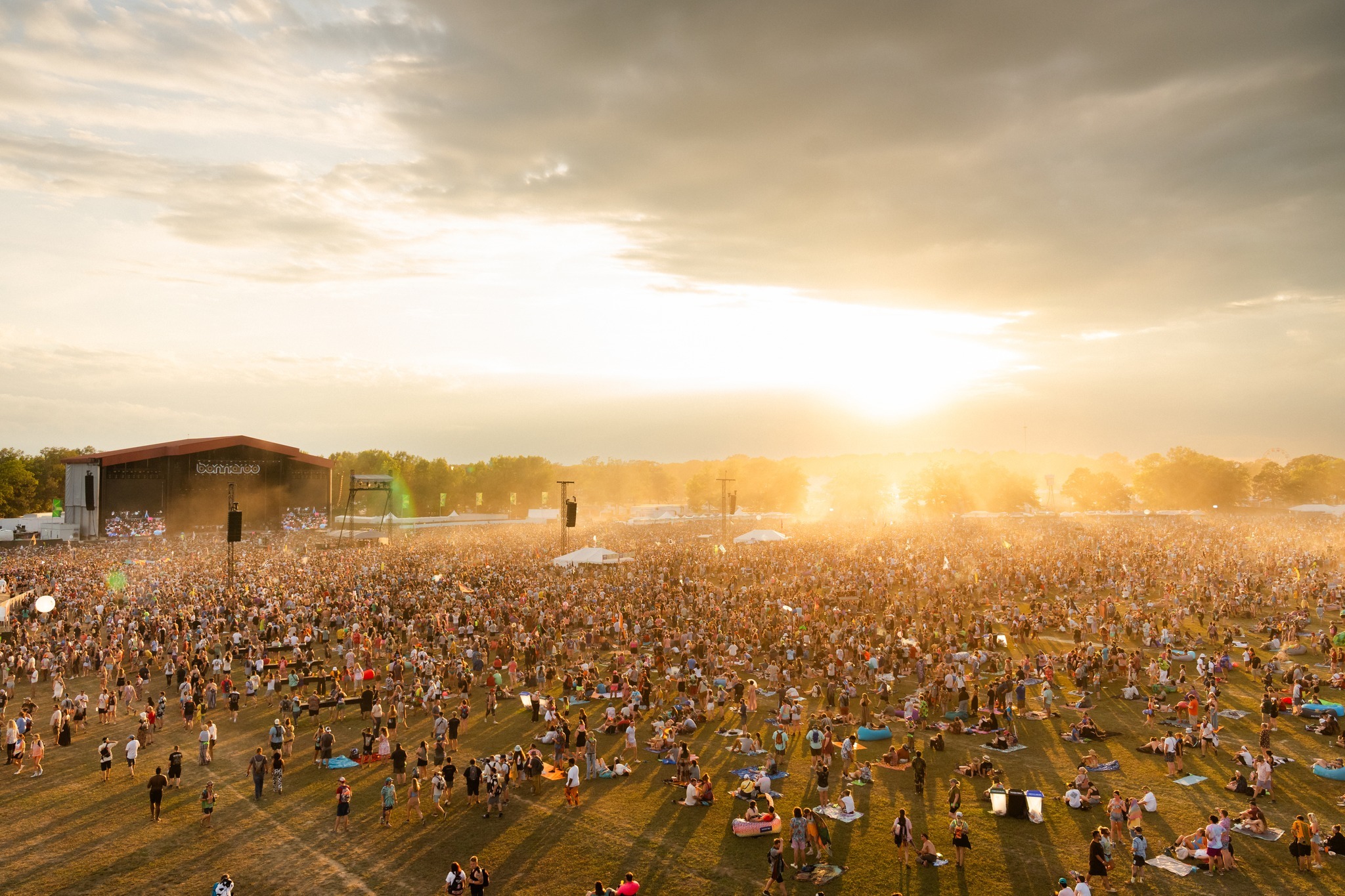This photograph captures an aerial view of a sprawling outdoor concert set in a vast field, teeming with thousands of people. The crowd extends from the bottom of the frame to the horizon, with high-density gatherings predominantly on the left and mid-right sections, particularly near the large stage in the top left. The stage, featuring a distinctive triangular roof reminiscent of a warehouse, is flanked by three substantial speakers mounted on crane-like structures, and numerous white tents are scattered nearby.

On the left side of the image, a line of buildings and a barn-like structure add a rustic touch to the scene, while tree lines frame both sides, reinforcing the natural venue. The attendees, dressed in summer attire, are seen standing closer to the stage while many sit or lie on blankets, tarps, and even inflatable pool toys further back, creating a relaxed, festival-like atmosphere as they spread out towards the bottom of the frame.

Dominating the sky is an interplay of dramatic dark and light gray storm clouds, with a large, radiant sun breaking through the gap between them. The sun’s vibrant white rays bathe the entire field in a golden, orange hue, casting a warm and almost ethereal glow over the scene below, enhancing the lively and dynamic ambiance of this outdoor gathering.